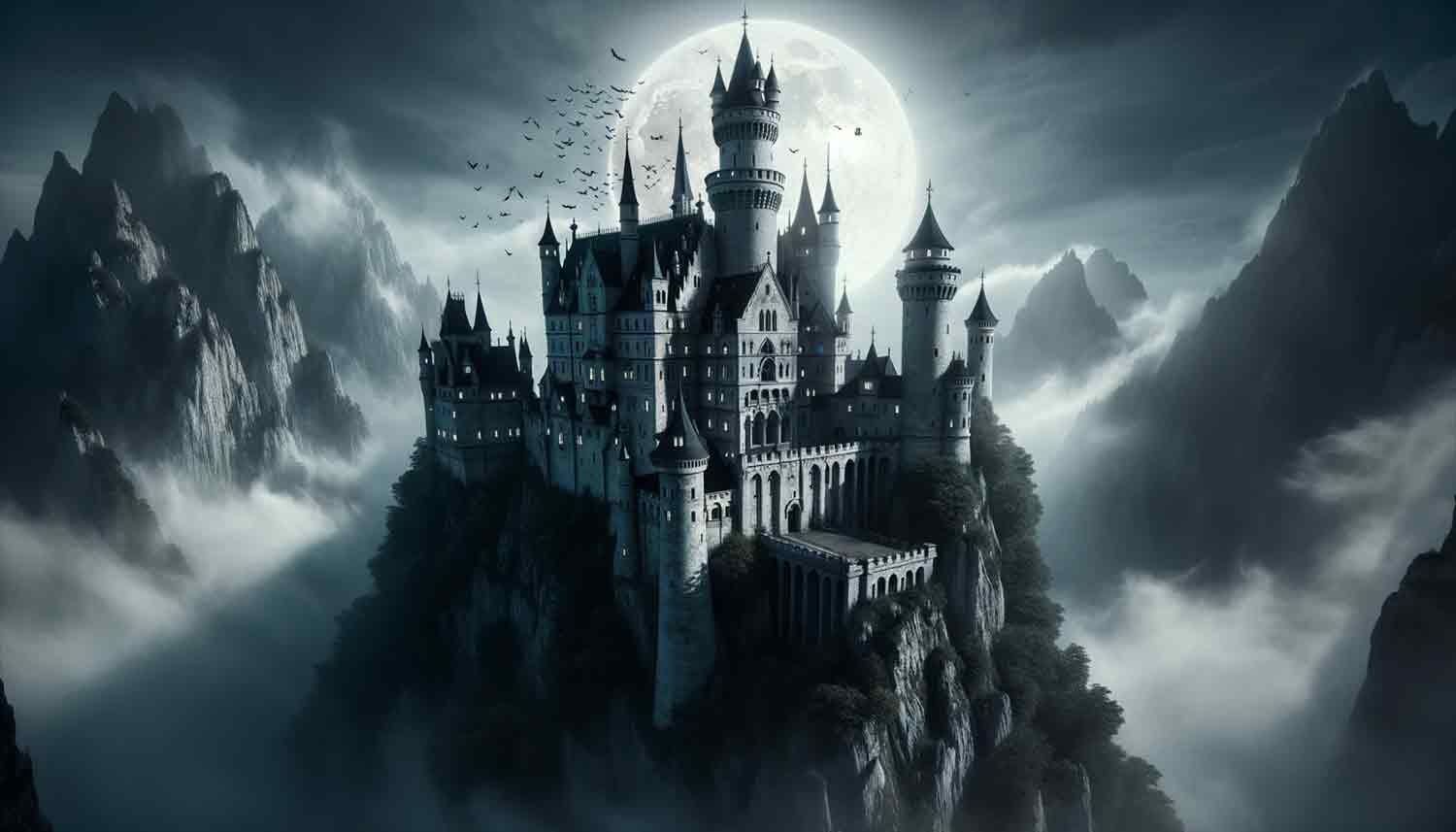The image is a computer-generated, highly detailed portrayal of a large, spooky castle perched atop a craggy mountain and surrounded by other jagged peaks under a dark, cloudy night sky. The entire scene has an eerie blue and gray color palette, heightening its mysterious atmosphere. Central to the composition, a massive, ancient castle with at least a dozen towering spires and turrets rises from the rocky summit. The highest tower is crowned with what might be a cross, while numerous lit windows glow warmly, contrasting the overall gloom. Behind the castle, a full moon, partially obscured by the tallest spire, casts a ghostly illumination over the landscape. Swarms of bats or black birds flutter in front of the moon, adding to the haunting vibe. Fog and mist weave through the mountain's crevices and hang low around the other peaks, creating a dreamlike haze that obscures the lower terrain. The setting is devoid of roads or paths, making one wonder how anyone could access such a lofty, secluded fortress. The entire image seems to be taken from a dramatic, cinematic shot, evoking a sense of gothic grandeur and mystery.